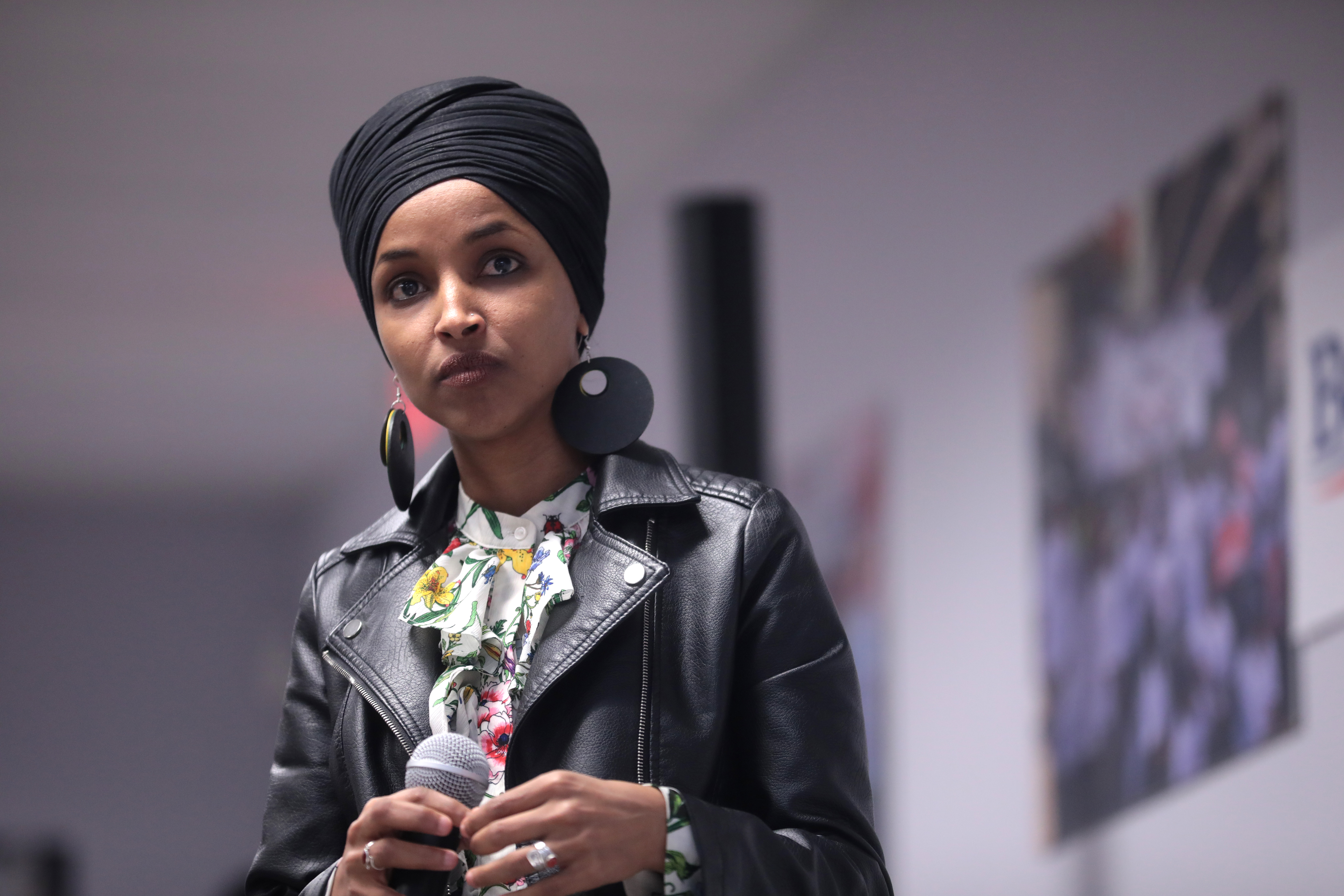In this indoor photo, Congresswoman Ilhan Omar stands slightly to the left of the center, gazing intently in front of her as she listens to someone speak. She is adorned in a black head wrap and large, round stone earrings that dangle elegantly. Her outfit includes a black leather jacket with buttons, rivets, and zippers, over a white floral blouse. Ilhan Omar is holding a microphone with both hands down below her mouth, the left hand meeting the right hand in front of her. Rings sparkle on each of her fingers. The background showcases a wall with colorful, yet indistinct, posters or banners, giving a sense of a vibrant setting. The color scheme in the photo includes black, white, gray, yellow, green, blue, light pink, and brown, suggesting a dynamic atmosphere likely at a speaking event.